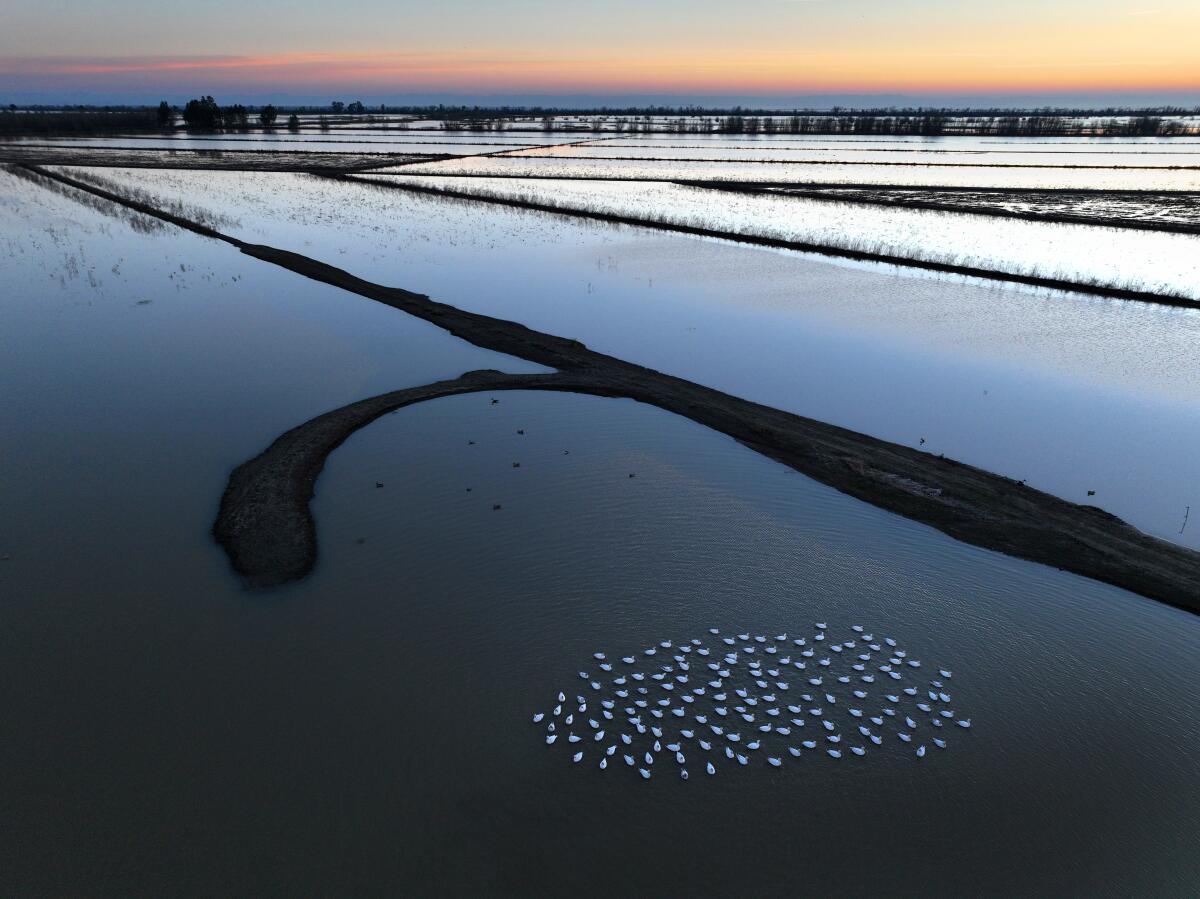This picturesque sunset scene captures a serene body of water, possibly a marsh or rice paddy field, bathed in the warm hues of dusk with a palette of blues, oranges, pinks, yellows, and corals. The horizon line, positioned at the top sixth of the image, showcases a stunning skyline with scattered trees that jut up from the islands in the background. The expansive water, reflecting the gentle light of the setting sun, features a multitude of island formations and pathways of land, suggesting a fluctuating water level.

In the foreground, a school of white birds—likely ducks—floats gracefully in a tight cluster. Each bird is oriented in the same direction, heads held high, creating a sense of unity and movement toward the forefront of the photo. The reflections and light rays dance across the water, enhancing the tranquil and picturesque atmosphere of this idyllic natural setting at dusk.